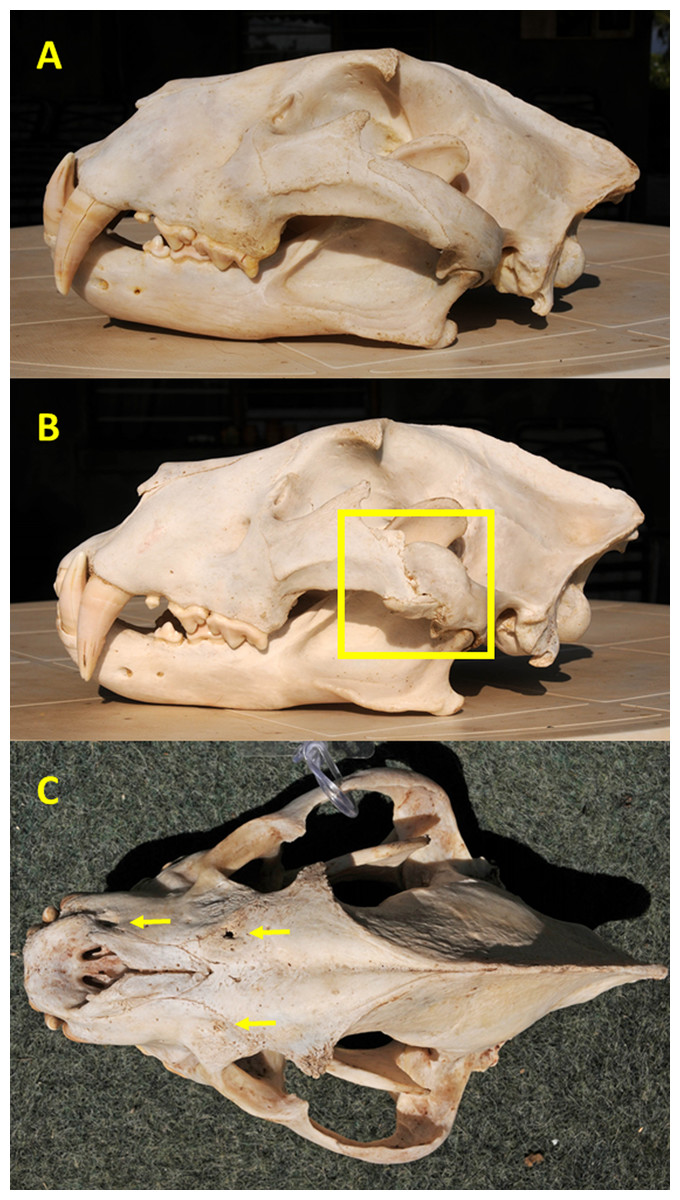This image showcases a detailed diagram of an animal skull, presenting it through three distinctly labeled views: A, B, and C. The skull, reminiscent of a large cat such as a saber-toothed tiger, features prominent large teeth and molars, with a distinctive sloped forehead leading to a point. Image A, positioned at the top, provides the cleanest side profile of the skull, highlighting the jaw and eye sockets. Image B, similar in angle to A, reveals a noticeable crack on one side of the head. Image C offers a top-down perspective, displaying additional cracks and holes along the skull, particularly around the nostrils and nose area. The skull appears white to off-white and is depicted on different backdrops: a brown table in A and B, and a green cloth or asphalt-like surface in C. This meticulous presentation suggests that the skull might belong to a prehistoric mammal, possibly a saber-toothed tiger, given its formidable jaw structure.